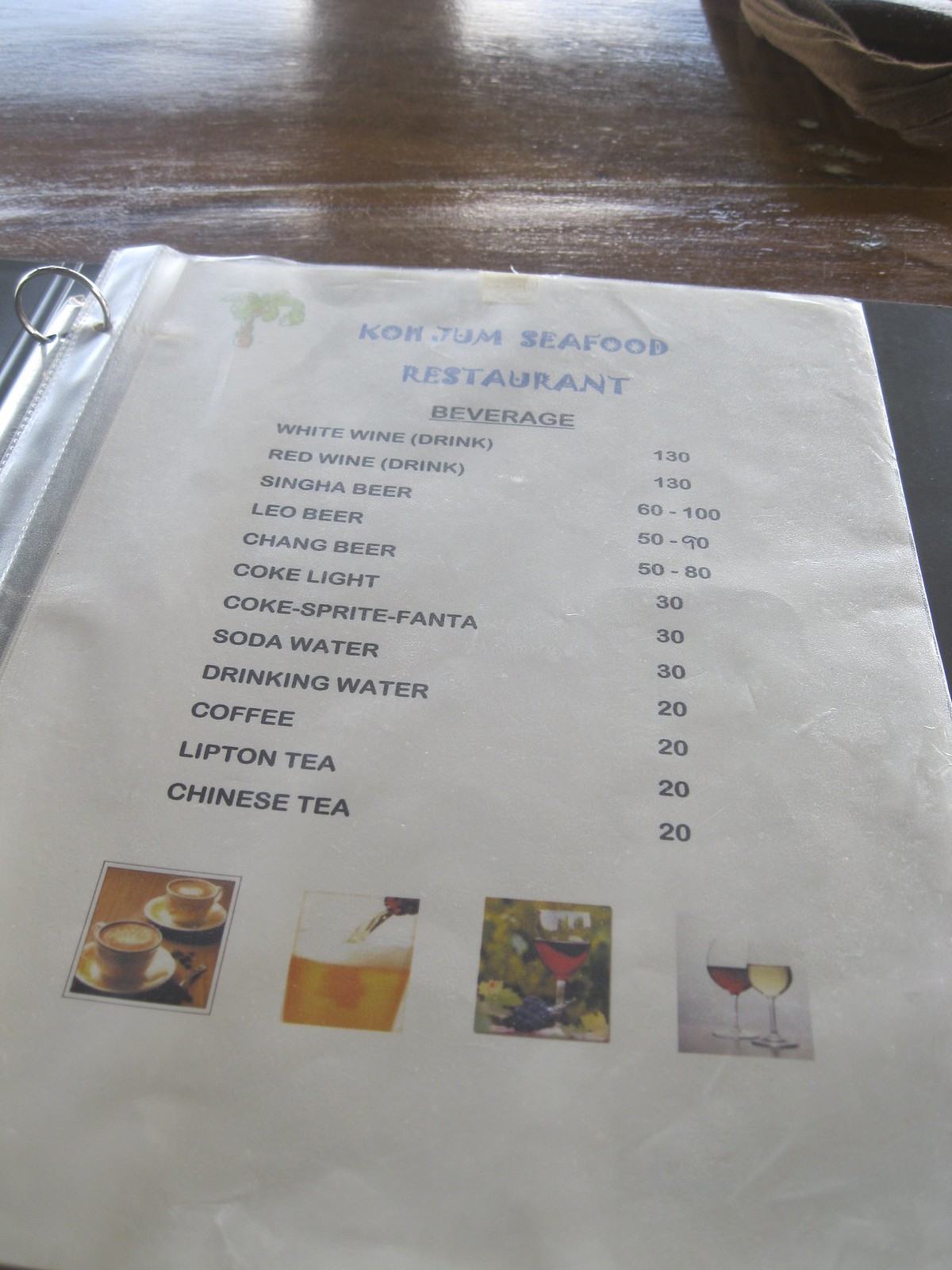This is a detailed photograph of a beverage menu at Konjum Seafood Restaurant. The menu is displayed on white paper, encased in a protective plastic sleeve, and placed within a black binder. The binder rings at the top left are silver. The menu prominently features the restaurant's name, "Konjum Seafood Restaurant," at the top, accompanied by a palm tree graphic on the top left corner. Below the title, "Beverage" is listed, followed by an extensive list of drink options with corresponding prices on the left and right sides respectively.

The beverage options include:
- White Wine: $1.30
- Red Wine: $1.30
- Singha Beer: $60-$100
- Leo Beer: $50-$90
- Chang Beer: $50-$80
- Coke Light: $30
- Coke, Sprite, Fanta: $30
- Soda Water: $30
- Drinking Water: $20
- Coffee: $20
- Lipton Tea: $20
- Chinese Tea: $20

At the bottom of the menu, there are four photographs depicting different drinks. From left to right, these images showcase a tea, a beer, a wine, and two wine glasses filled with red and white wine. The menu rests on a wooden table, completing the setting for this elegant display at the seafood restaurant.